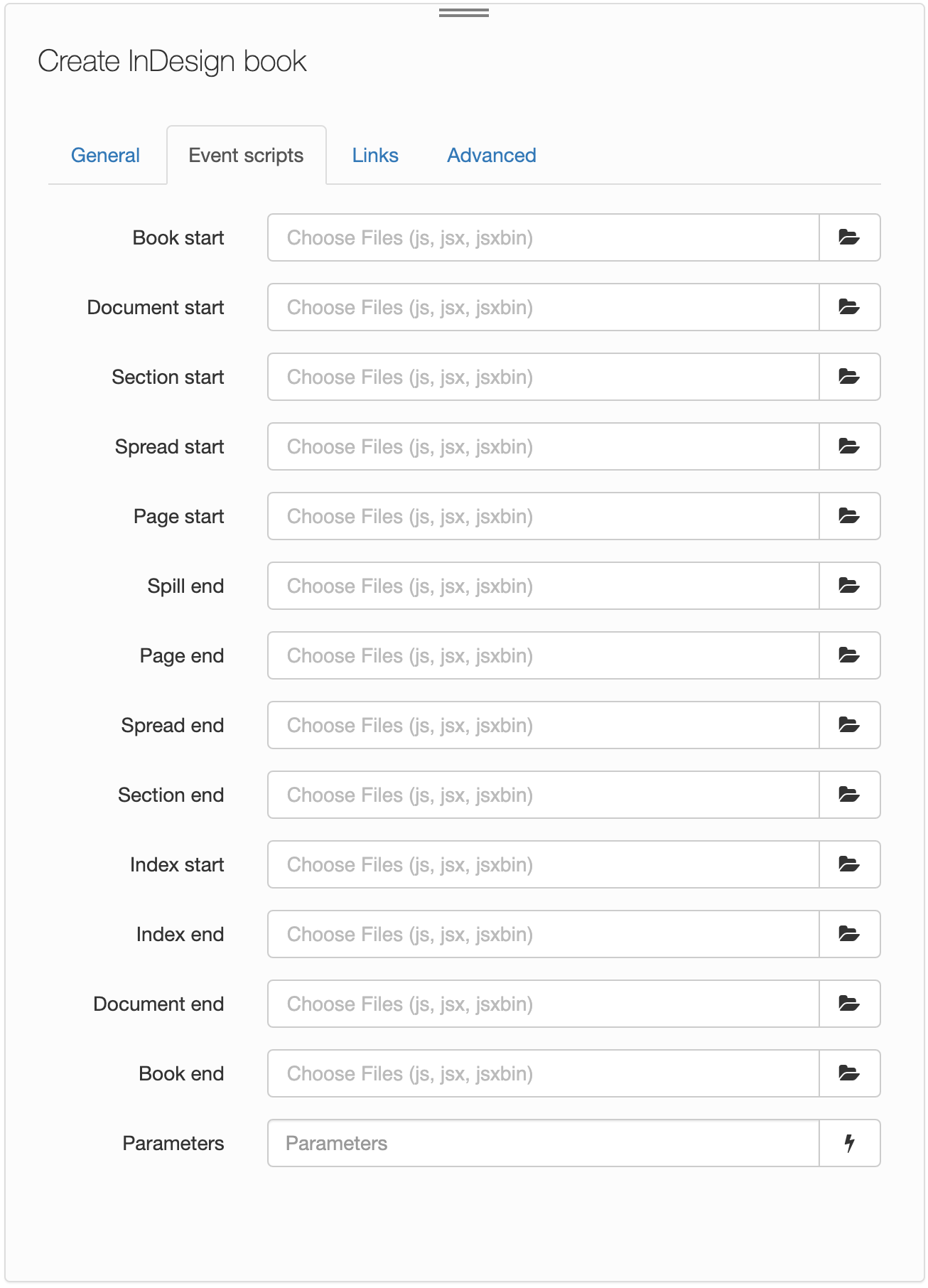The image captures the interface of a design software tool with a light gray background. At the top of the screen, it prominently displays the option to "Create in Design Book." Below this header are four clickable tabs: "General" in blue, "Event Scripts" in black, "Links" in blue, and "Advanced" in blue. The "Event Scripts" tab is selected, highlighted by a horizontal line running across the top and bottom of the tab.

Within the "Event Scripts" tab, there's a structured layout featuring a column on the left, a central box, and a "File" button on the right. Each section in the central box offers a dropdown menu labeled "Choose File" with options like JS, JSX, JSX BIN.

The left column lists various script trigger points, arranged from top to bottom as follows: "Book Start," "Document Start," "Section Start," "Spread Start," "Page Start," "Spill in," "Page End," "Spread End," "Section End," "Index Start," "Index End," "Document End," "Book End," and "Parameters."